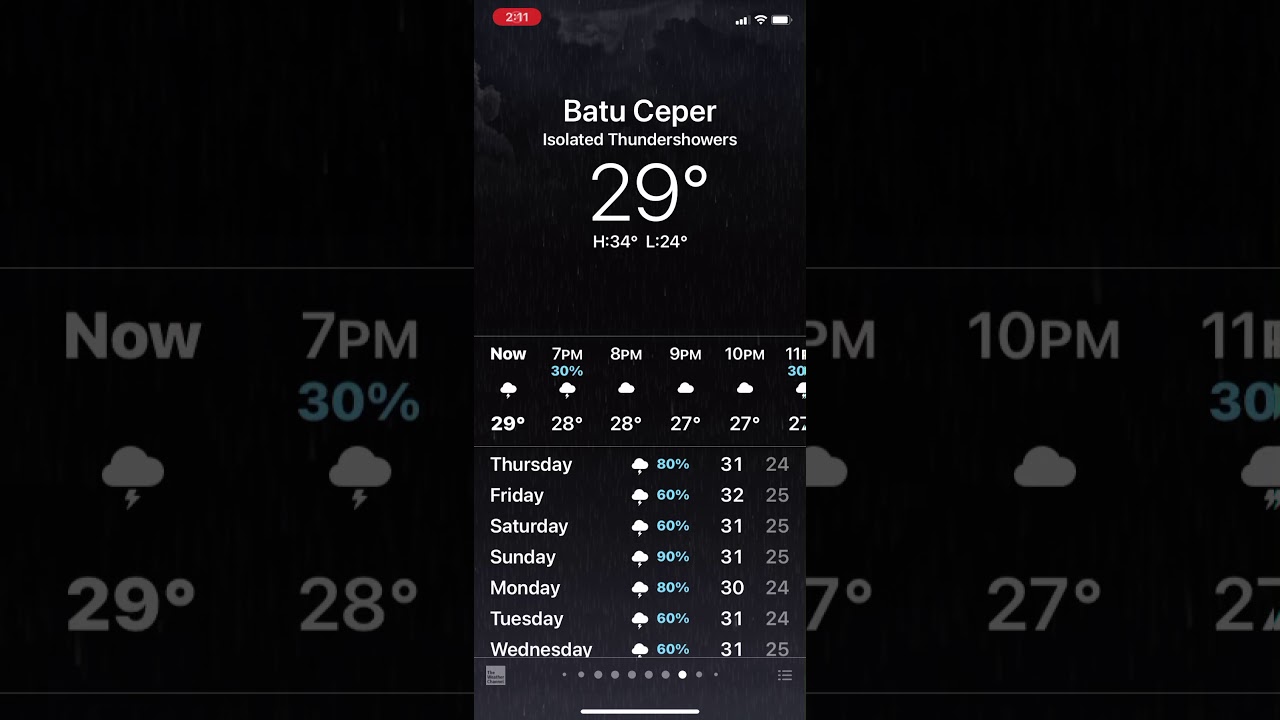The screenshot displays a weather forecast on a cell phone screen at 2:11 (AM/PM unspecified). The phone shows a strong signal with three out of four bars for cellular reception, full Wi-Fi strength, and an almost fully charged battery status, as indicated in the upper-right corner. The forecast location is BATU CEPR. The current conditions are described as isolated thunderstorms with a temperature of 29°C; the high for the day is expected to reach 34°C and the low to drop to 24°C.

The detailed hourly forecast follows:
- 2:11: 29°C with isolated thunderstorms.
- 7 PM: 30% chance of thunderstorms, 28°C.
- 8 PM: Cloud cover, 28°C.
- 9 PM: Cloud cover, 27°C.
- 10 PM: Cloud cover, 27°C.
- 11 PM: 30% chance of rainstorms, 27°C.

The extended forecast indicates:
- Thursday: Thunderstorms with an 80% chance, high of 31°C, low of 24°C.
- Friday: 60% chance of thunderstorms, high of 32°C, low of 25°C.
- Saturday: 60% chance of storms, high of 31°C, low of 25°C.
- Sunday: 90% chance of storms, high of 31°C, low of 25°C.